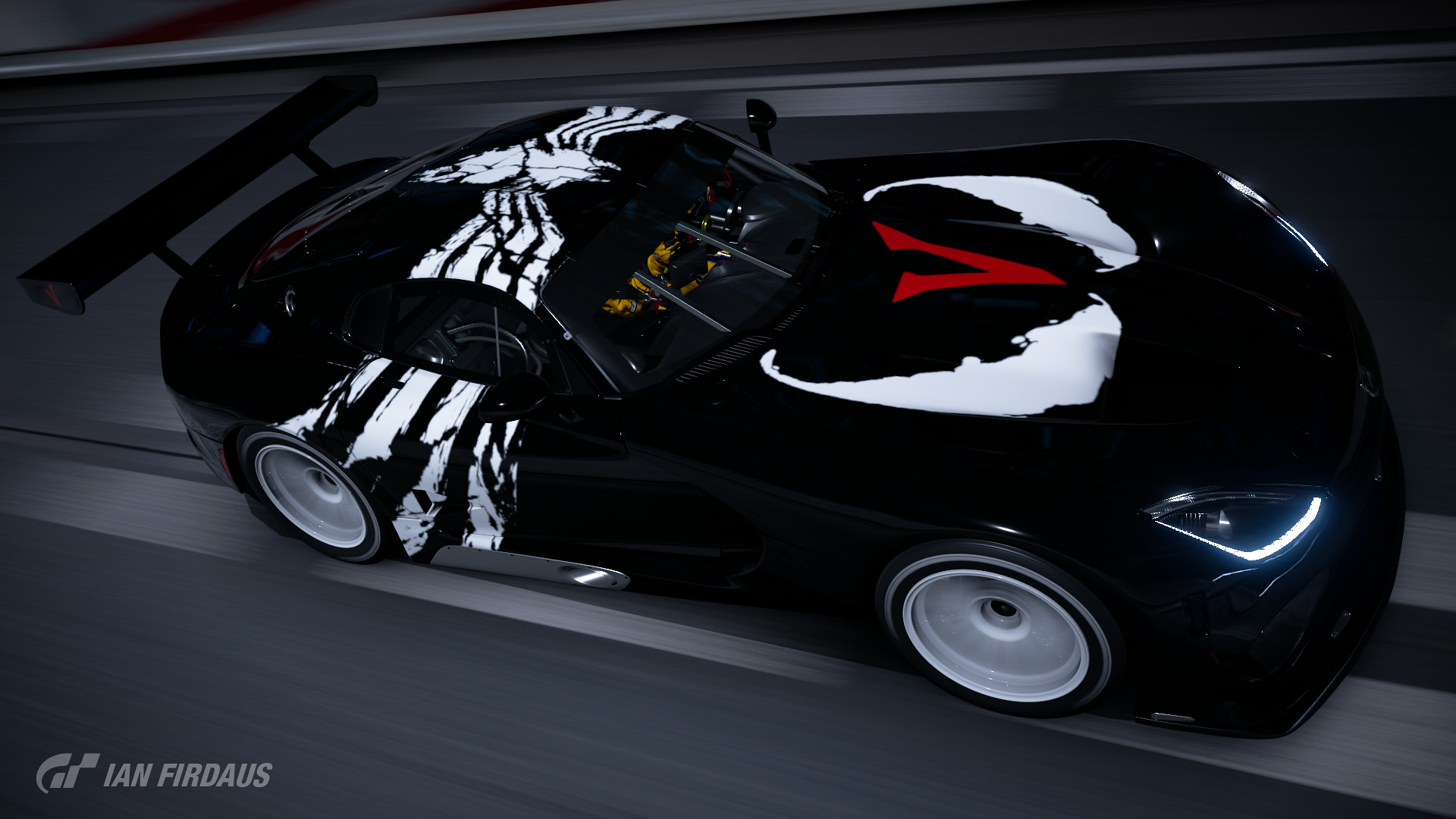This image captures a modified black sports car, prominently positioned in the center of the scene, possibly on a closed professional track at nighttime. The setting is outdoors, featuring an asphalt road with a blurred wall in the background, suggesting high speed. The photograph incorporates various shades including black, white, red, tan, brown, gray, and silver. The car, resembling a Chevrolet Corvette with modifications that give it a similar appearance to a Dodge Viper or even the Batmobile, is adorned with distinctive white designs that resemble the Spider-Man villain Venom. Prominently, a large red 'V' is displayed on its hood, with reflective elements hinting at a white ceiling above. The car's substantial tail fin and white rims further accentuate its striking appearance. The image is quite dark, with the car's headlights activated, emphasizing its aggressive stance. In the bottom left corner, the text "Ian Ferdows" or "Ian Firdos F-I-R-D-A-U-S" is visible, accompanied by a GT logo.